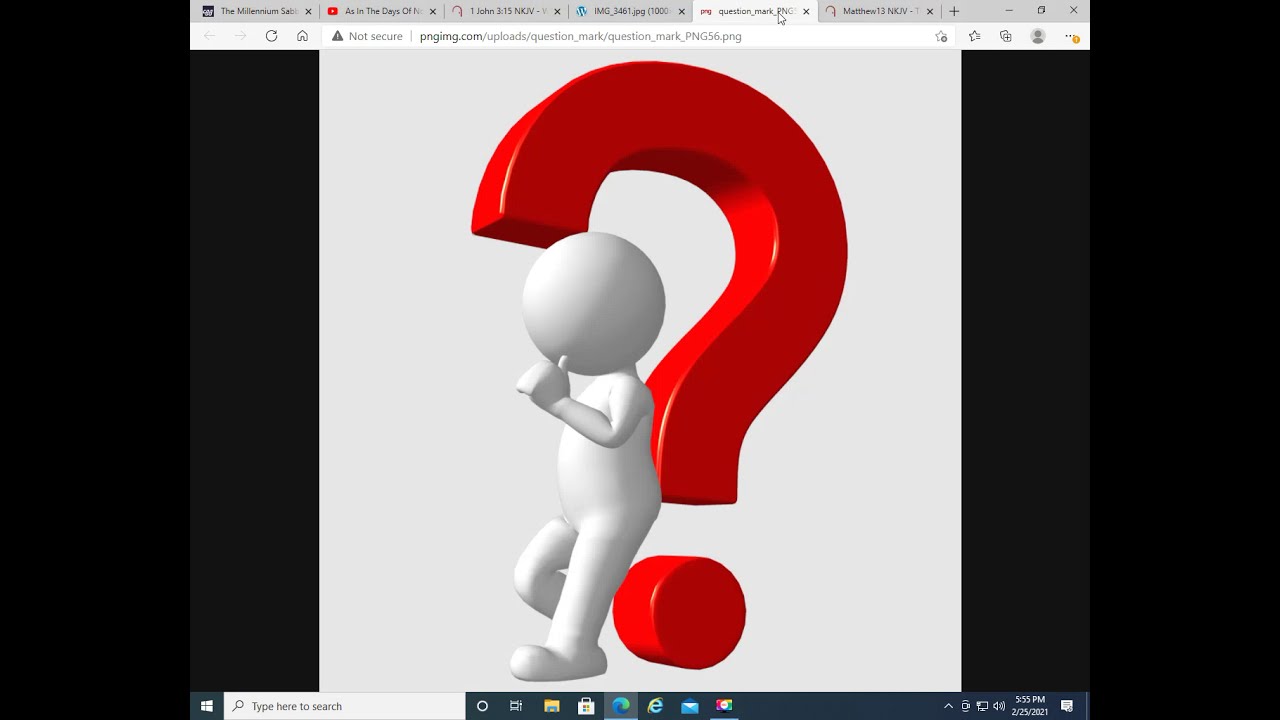The screenshot depicts a desktop environment, likely from a Windows device, as evidenced by the taskbar at the bottom displaying familiar icons such as Internet Explorer, Outlook, Firefox, and a search bar, along with the time, which reads 5:55 p.m. on February 25th, 2021. The main focus of the image is a web browser window with numerous tabs open, including YouTube, a news site, and pages labeled "John 3:15" and "Matthew 13," suggesting some religious content.

The active tab shows a webpage with the URL “pngimg.com/uploads/questionmark/questionmark-mark.png56.png.” Central to the browser window is a white background featuring a three-dimensional, shiny red question mark. Leaning against the question mark is a white, bubble-like stick figure with a round head and simple, featureless body, giving the figure a somewhat neutral or emotionless appearance. The image is framed by black vertical bars on the left and right sides, further emphasizing the main content. The overall background color of the webpage appears to be a very light gray.